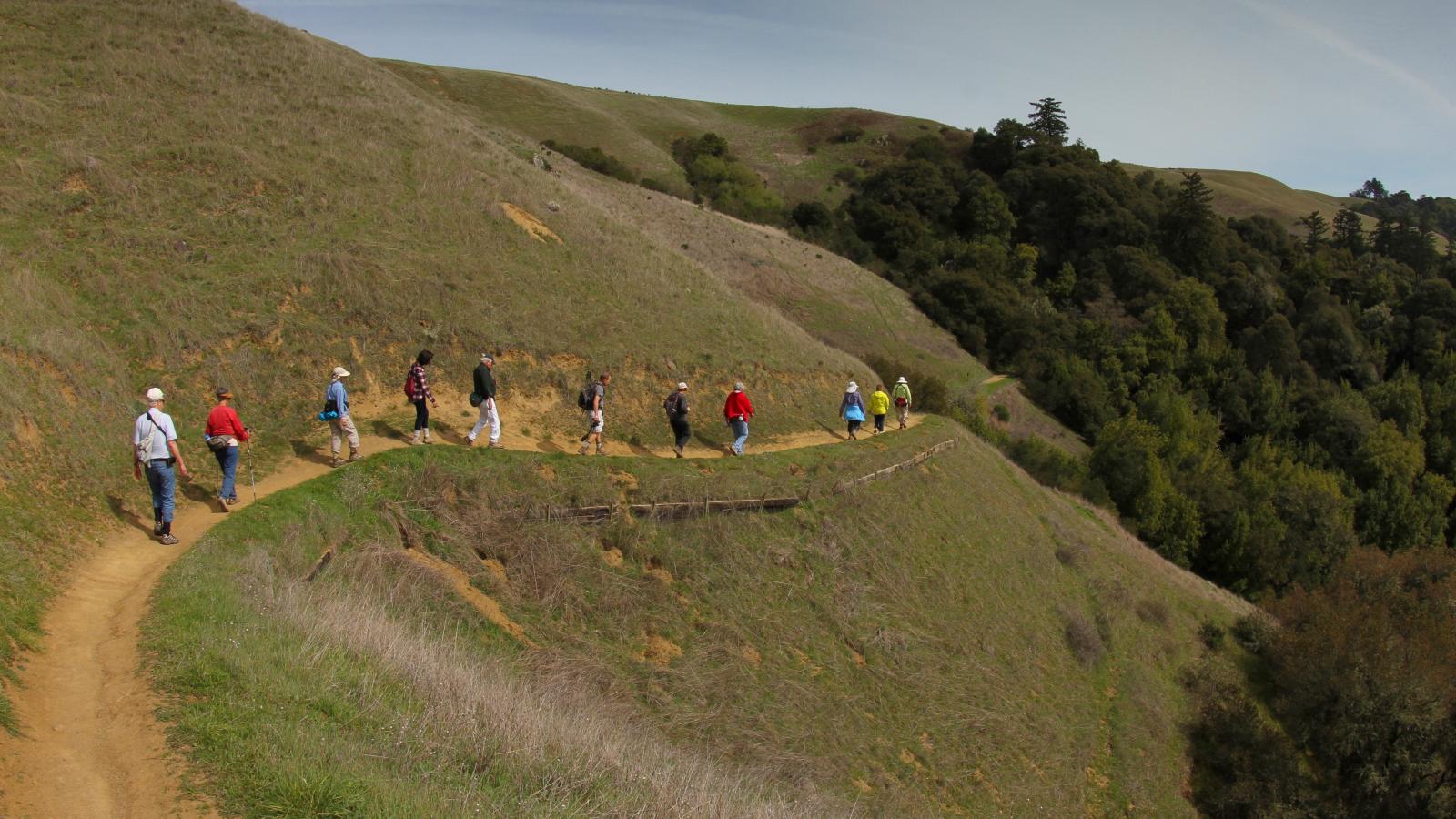The image depicts a group of 11 hikers, consisting of various ages including some elderly individuals and a child, traversing a dusty brown trail that winds through greenish-brown hills. The hikers, adorned in brightly colored clothing and carrying backpacks, are arranged in a single file line, evenly spaced apart, likely for safety and cohesion. The trail is situated along the edge of the hills, with safety rails in place to prevent erosion. To the right side of the picture, dense clusters of trees are visible, while the left side displays more barren, grassy terrain. The background showcases a pale blue, cloudless sky, enhancing the vividness of the hikers' attire. The image captures the hikers' journey through these rolling, grassy hills as they approach a forested area, underscoring the natural beauty and the structured organization of their expedition.